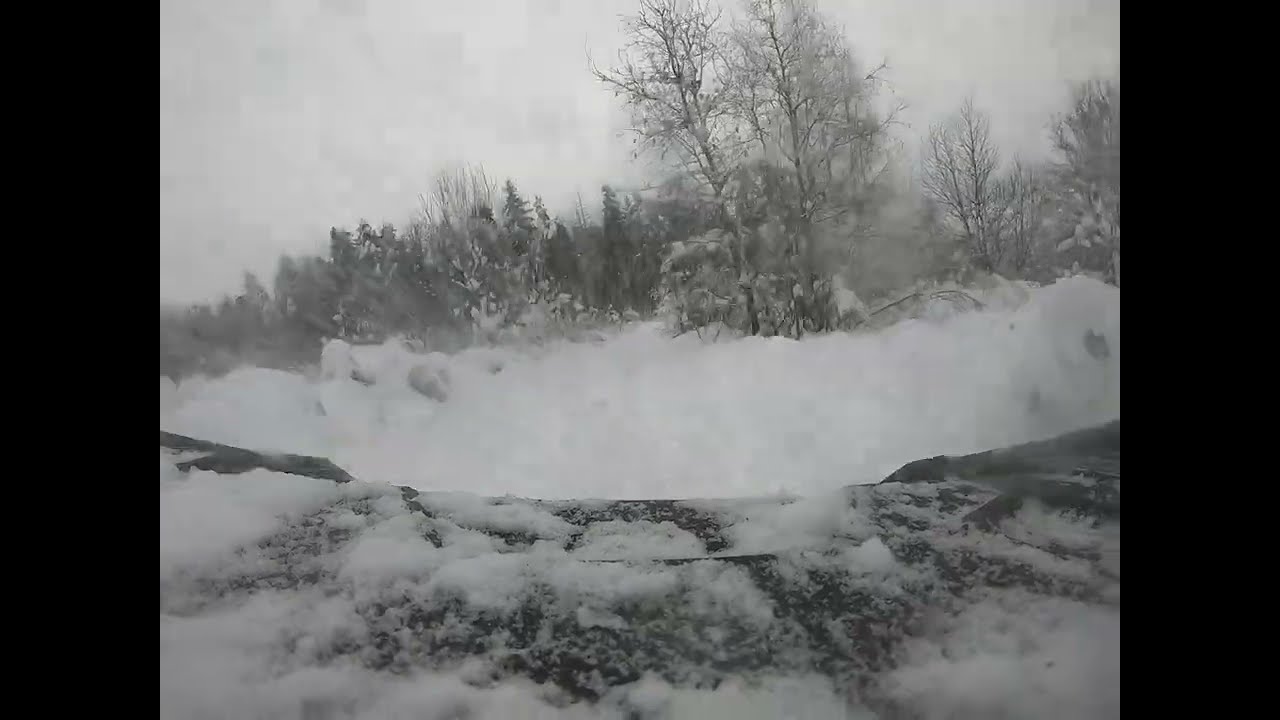A snowy, icy landscape captured in a pixelated and blurry photograph framed by two vertical black bars on the left and right edges. The daytime sky above is a dull gray, devoid of clouds, adding to the cold ambiance. A large pile of snow covers a rocky ledge in the foreground, where a snow-covered scoop or shovel is visible, seemingly pushing the snow towards the barren trees in the background. The landscape is dotted with leafless trees, with an occasional green pine tree standing out. The surrounding snowy expanse appears both cold and desolate, resembling a wintry canyon filled with white snow. The heavily distorted image might have been taken by a ring or door camera, further contributing to its indistinct details.